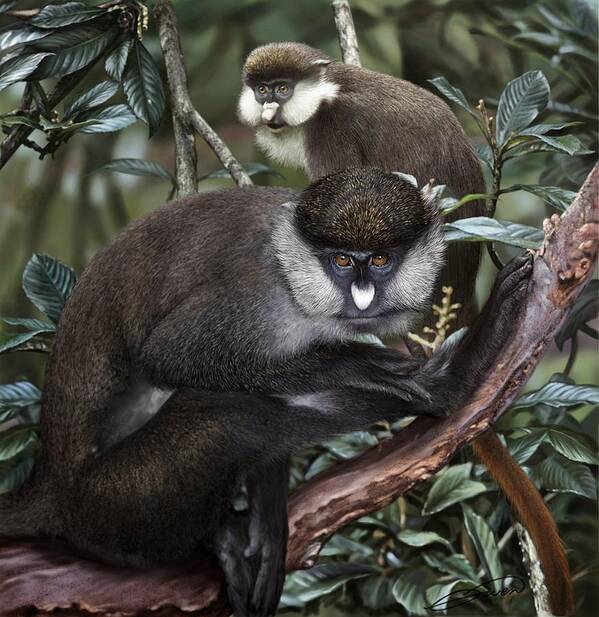In this detailed color photograph, two monkeys are perched on tree branches amid an abundance of deep, glossy green leaves. The larger monkey, positioned in the foreground, gazes directly at the camera with striking bronze-colored eyes. Its face is predominantly black, accented by a white, furry beard and a distinctive white nose with a black tip. This monkey's body is cloaked in a rich, chocolate brown fur with darker black patches, and it has a long, lighter brown tail that dangles from the branch. One of its paws is visibly resting on the branch.

The smaller monkey, sitting just behind the first, is angled slightly to the left with its mouth open. It features similar facial markings, including a black face, white nose, and additional white fur around its cheeks and chest. Both monkeys' noses have a white tip and dark top. Their small ears and bushy hair add to their unique appearance. The background of the image is dominated by the dark green leaves, which frame the edges of the photograph and enhance the natural, tropical atmosphere of this scene.